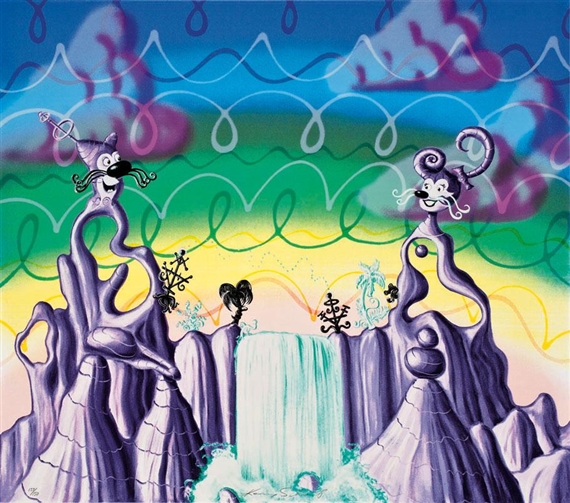This square digital artwork features a striking, abstract landscape with a multi-colored sky transitioning from dark bluish tones at the top, through gray-purple clouds, into deep green, and finally into bright yellow, forming curved bands resembling a rainbow. The sky is adorned with numerous squiggly lines in varying shades of gray, blue, green, and yellow. Below this dynamic sky, two surreal, purple mountain peaks each embody a whimsical, cartoonish character. On the left, a male character with a big black nose, whiskers, and an antenna-like feature on his head, smiles toward the right. On the right, a female character with similar features but adorned with long, curled purple hair and white whiskers, gazes back at him. Their ears appear to be morphing into tentacle-like shapes. Positioned between them is an off bluish-green abstract waterfall cascading down the mountains. Adding to the surreal nature, the left side of the scene features a black palm tree, while a light blue palm tree mirrors it from the right. Throughout this imaginative piece, small rounded shapes in pink, orange, and purple, as well as meandering black lines, punctuate the landscape, enhancing the fantastical essence of the artwork.